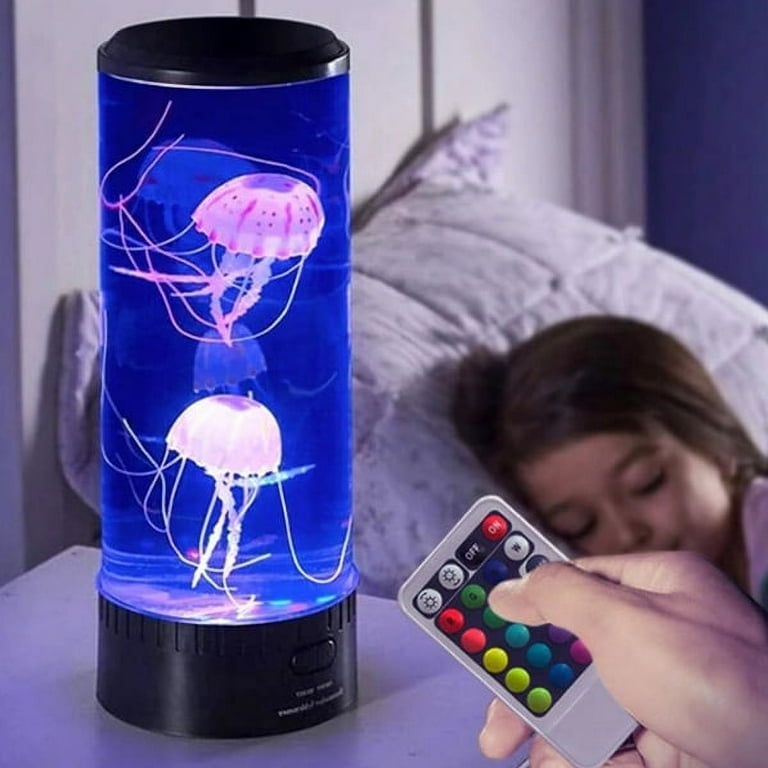The image shows a detailed advertisement for a jellyfish-themed, color-changing LED lava lamp, ideal for a child's bedroom. The lamp has a sleek design with a black base and cap, and it features multiple, holographic-like jellyfish that appear to swim in a blue liquid. The lamp can change colors via a remote control, which is visible in the lower right-hand corner being held by a hand. The remote offers various settings, including an on/off switch, brightness adjustments, and different color options. At least six jellyfish are seen, with prominent purple and pink hues. The background has an ambient sea-like blue color, adding to the underwater illusion. A little girl is peacefully sleeping in her bed, her head resting on a white pillow, with white and blue walls surrounding her. The lava lamp is positioned on her bedside table, softly illuminating her space.